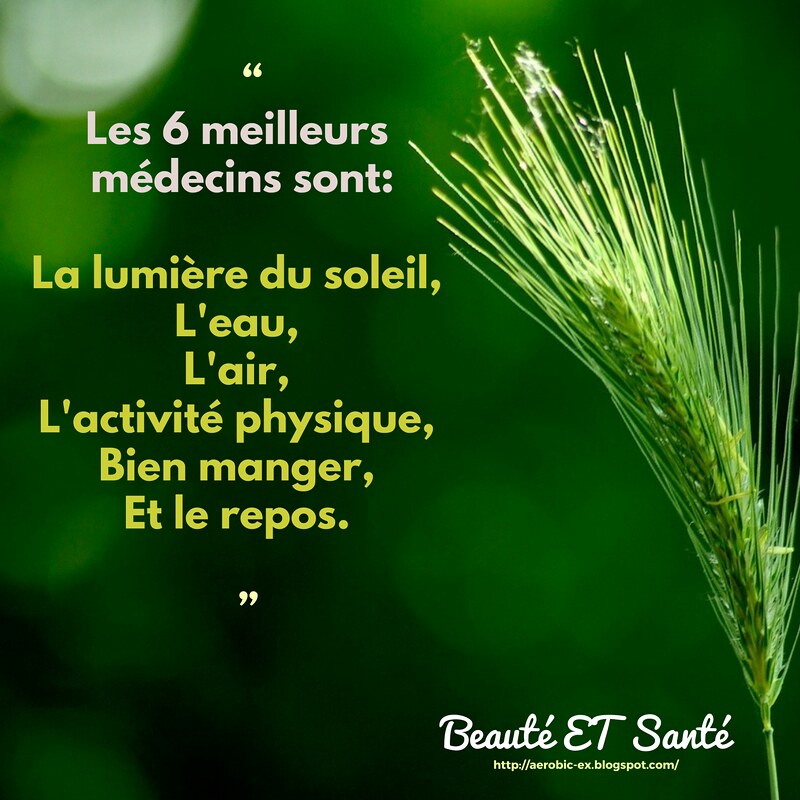The image features a muted green background with a bokeh effect. From the bottom right corner, a green stem extends upwards, adorned with a cluster resembling pine needles, reminiscent of a fern or evergreen tree. The text on the poster is in French. In the upper left corner, white text in quotation marks reads "Les 6 meilleurs médecins sont:". Following this in yellow text are the words "la lumière du soleil, l'eau, l'air, l'activité physique, bien manger et le repos." In the bottom right corner, white cursive text reads "Beauté et Santé". Additionally, a website in white text, "aerobic-ex.blogspot.com", is located at the bottom of the poster. The overall color theme of the image is primarily green with accents of yellow.